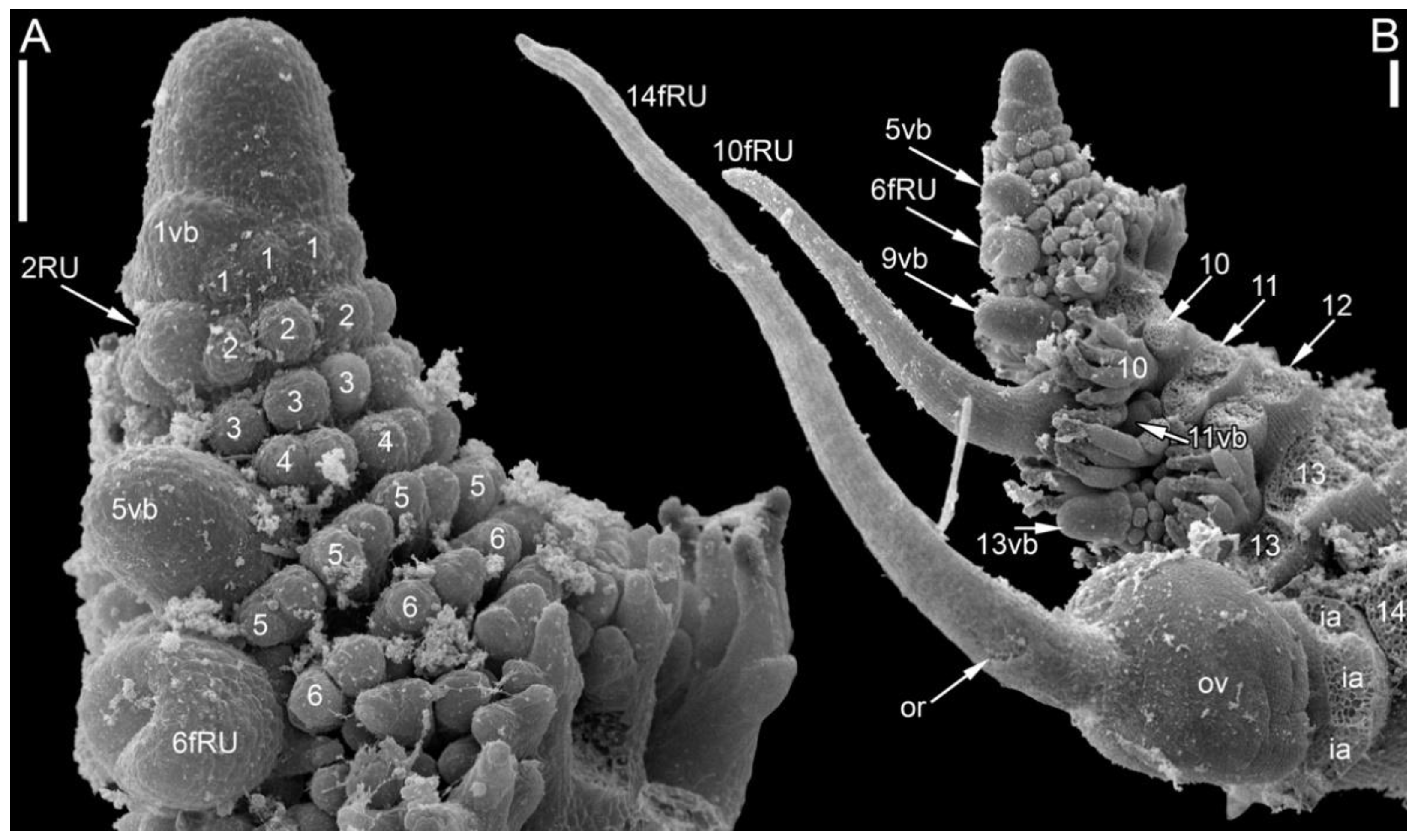This close-up, black-and-white image, possibly captured with a scanning electron microscope, features a detailed view of a complex, sea-like object that resembles algae or coral with numerous polyps. The object is divided into two labeled sections; the top-left corner is marked 'A', and the top-right corner is labeled 'B', each with corresponding numeric labels for various parts of the object. The labels include a combination of numbers and letters: on the left (A) side, rows are marked 1 through 6, and on the right (B) side, the numbering includes IA, 10, 11, 12, 13, and 14. Additionally, specific sections are labeled with alphanumeric codes like 5BB, 6FRU, and 2RU. The right side of the object extends into what appear to be tentacle-like structures, enhancing its resemblance to underwater flora or fauna. Arrows and white lines point to specific areas, adding to the scientific and technical nature of the image, which seems to be a part of a detailed scientific or medical study.